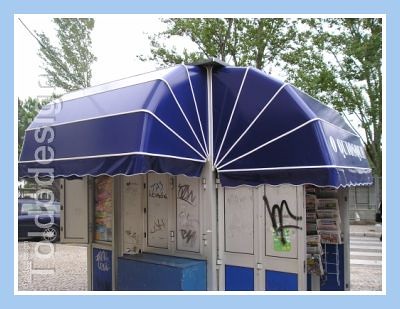The image depicts a vibrant, blue-awning-topped newsstand or small street booth positioned on a street corner. The structure features a white and blue door with visible graffiti consisting of black characters. The booth is stocked with an assortment of magazines, newspapers, and snacks, and there are white place cards for posters at the bottom. In the background, the scene is set against a cloudy sky with patches of blown-out areas due to brightness. Adjacent to the stand, a blue car is parked perpendicular, and there's a wide stone sidewalk offering pedestrian space. Green-leaved trees with brown branches can be seen, adding a touch of nature to this urban snapshot. Additionally, metal rods secure the awning, emphasizing the structure's durability. Displays and plaques adorn the booth, and part of a label reading "TAL DEDOS" or "Tolo Design" is visible. The photograph is framed with a blue border and a white matte, highlighting the color-rich, lively outdoor setting.